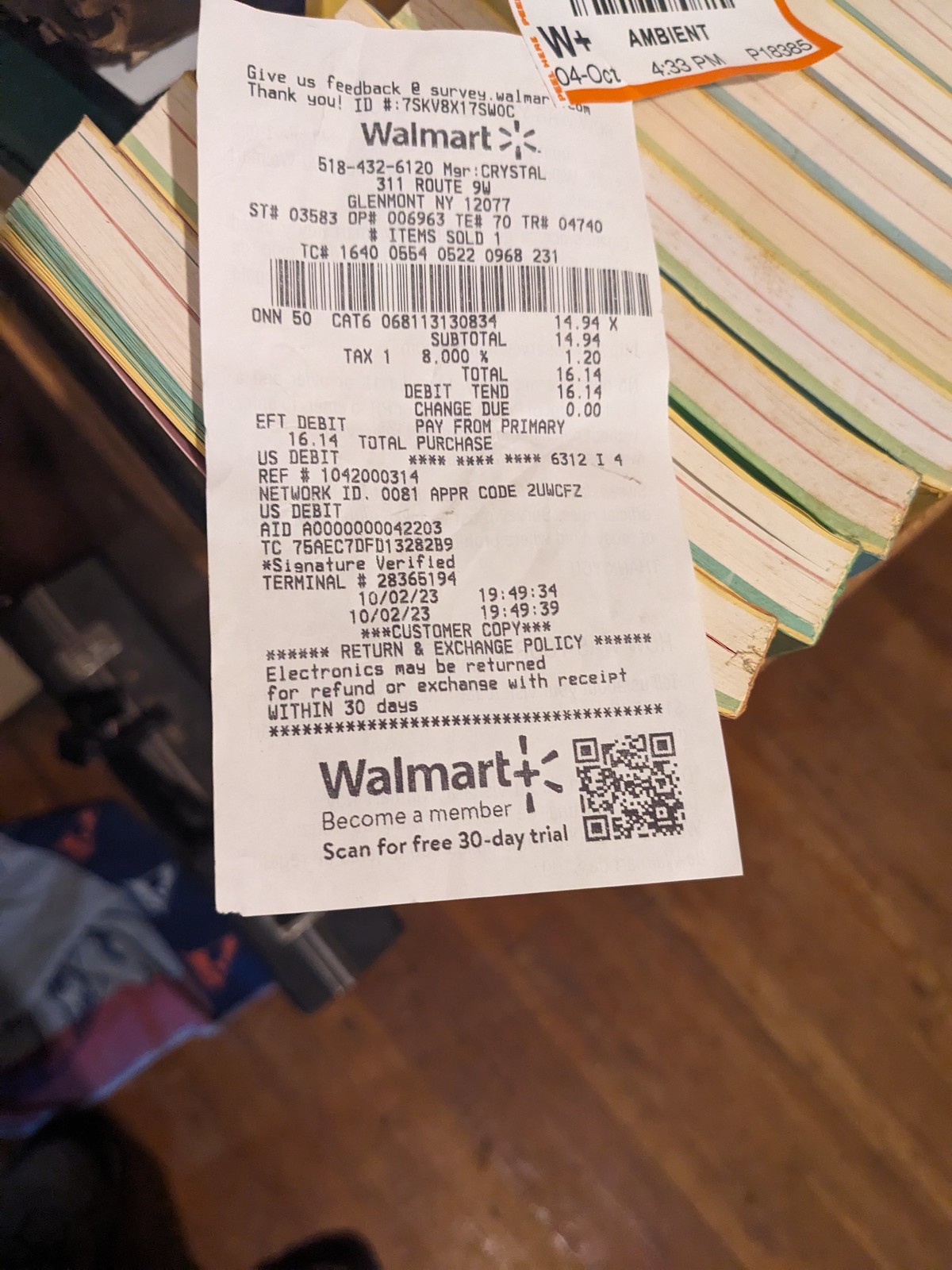A close-up image capturing a white, rectangular receipt from Walmart prominently displayed against the background of a bookshelf and wooden floor. The receipt, issued from a Walmart located in Glenmount, New York, features the store's name at the top, followed by detailed information about a recent purchase, presented in black text and numbers typical of a standard receipt. Barcodes conveying specific details about the transaction and store appear intermittently along the paper. Highlighted at the bottom is a QR code accompanied by text inviting customers to "scan for a free 30-day trial." The receipt is adorned with a small white sticker featuring an orange border, adding a pop of color. In the background, several books are visible, their spines partially obscured, hinting at a cozy, home-library setting. The entire scene is grounded by the hardwood flooring beneath.